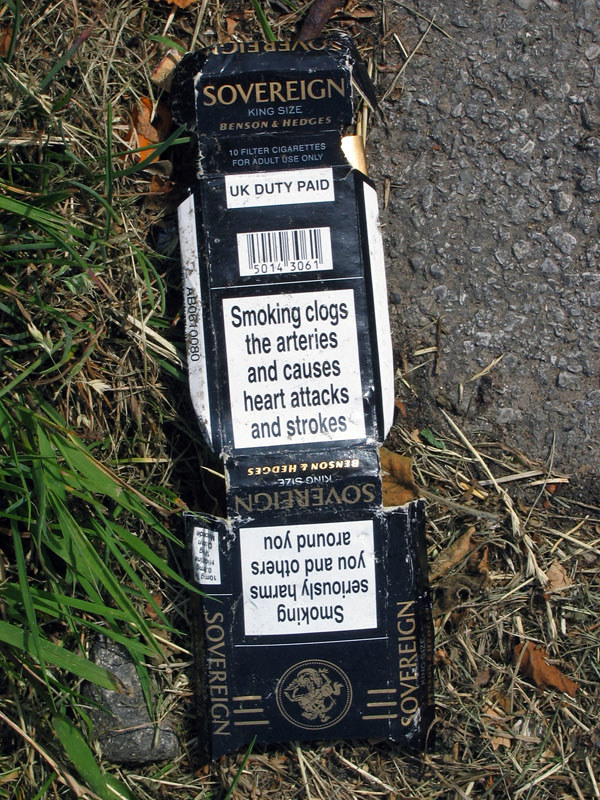This detailed color photograph, taken outdoors, captures a close-up view of a torn and flattened black cigarette package lying on the ground where a grassy area on the left meets a patch of black and gray asphalt on the right. The cigarette box, which appears unfolded and spread out, is surrounded by a mix of green long grass, dead grass, and leaves. The brand name "Sovereign" is prominently displayed at the top in gold lettering, followed by "King Size" and "Benson and Hedges" underneath. The package indicates it contains "10 Filter Cigarettes for Adult Use Only" and notes "UK Duty Paid." Beneath a barcode numbered 5014 3061, a white warning box with black text reads, "Smoking clogs the arteries and causes heart attacks and strokes." Another warning, "Smoking seriously harms you and others around you," is also visible. The text on the package is somewhat jumbled and upside-down due to its damaged state, but the distinctive gold and white labeling remains clear.